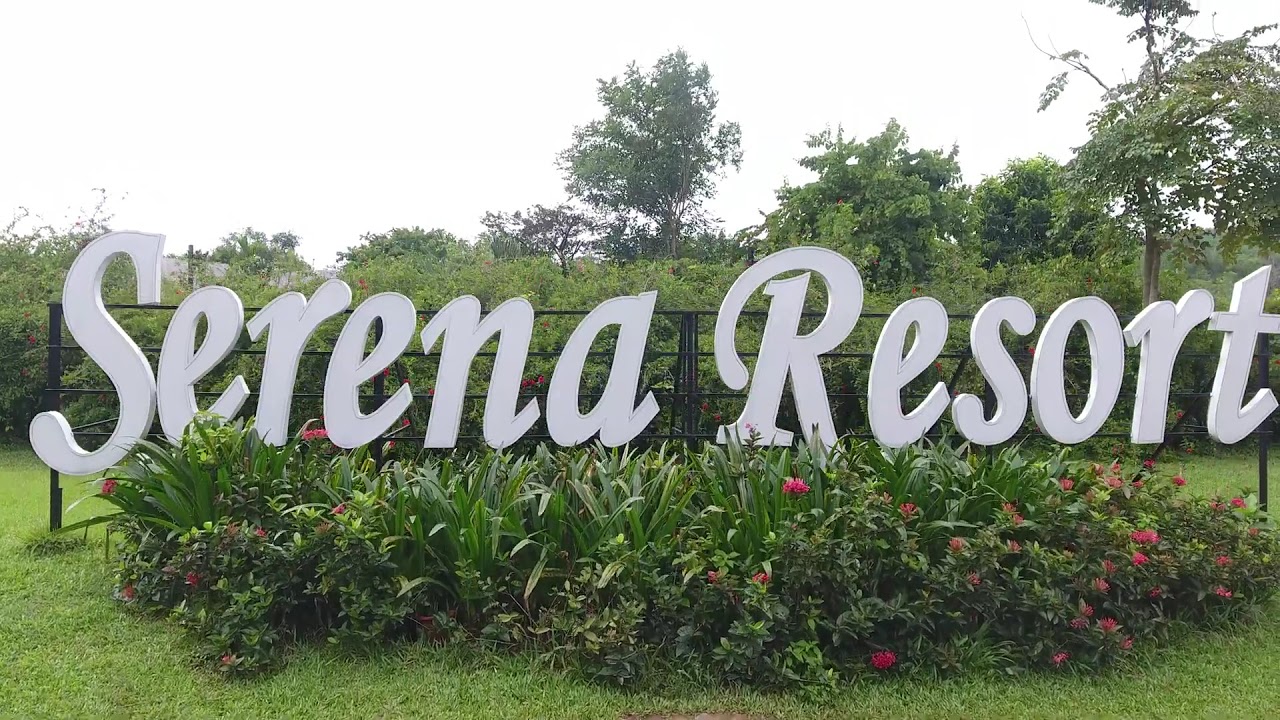This color photograph, taken in landscape orientation, captures the entrance signage to Serena Resort. The sign, featuring large white letters in a swash, slightly italic typeface, reads "Serena Resort" and spans across the entire width of the image. These letters are mounted on a black wireframe fence. Below the sign is a circular island of ornamental plants, including vibrant green grasses and red flowers on the right side, with a few additional pink or red flowers on the left side. The background showcases a line of shrubbery and taller green trees in the top right corner, enhancing the lush, inviting atmosphere of the resort's entrance.